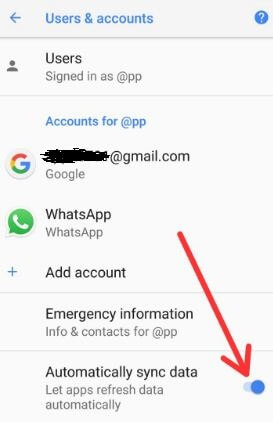This screenshot, taken from a mobile phone, displays the "Users and Accounts" settings page. At the top left corner, there's a blue back arrow, and at the center of the top banner, "Users and Accounts" is written in blue text. On the top right corner, there's a blue circle icon with a white question mark, likely for help or information.

Beneath the top banner is a light gray separator bar. The first section below the separator shows a person icon with the text "User signed in with apps." There's a blue hyperlink reading "Accounts for app." Below this, there's a Gmail account entry represented by the recognizable Gmail "G" logo, with the email address obscured except for the "@gmail.com" domain. Under this there’s a "Google" label, indicating the type of account.

Further down, the WhatsApp section is displayed, with the green WhatsApp logo featuring a phone icon inside it, followed by the text "WhatsApp" twice, signifying the logged-in user’s WhatsApp account.

Subsequent to this is a plus icon accompanied by the text "Add account," suggesting an option to add another account. Below, there's a section titled "Emergency information, info and contacts for app."

At the bottom is the "Automatically sync data" section with a brief description: "lets apps refresh data automatically." A blue toggle button next to this description indicates that auto-sync is currently enabled. A large, red, seemingly photoshopped arrow points directly at the activated toggle button, emphasizing it.